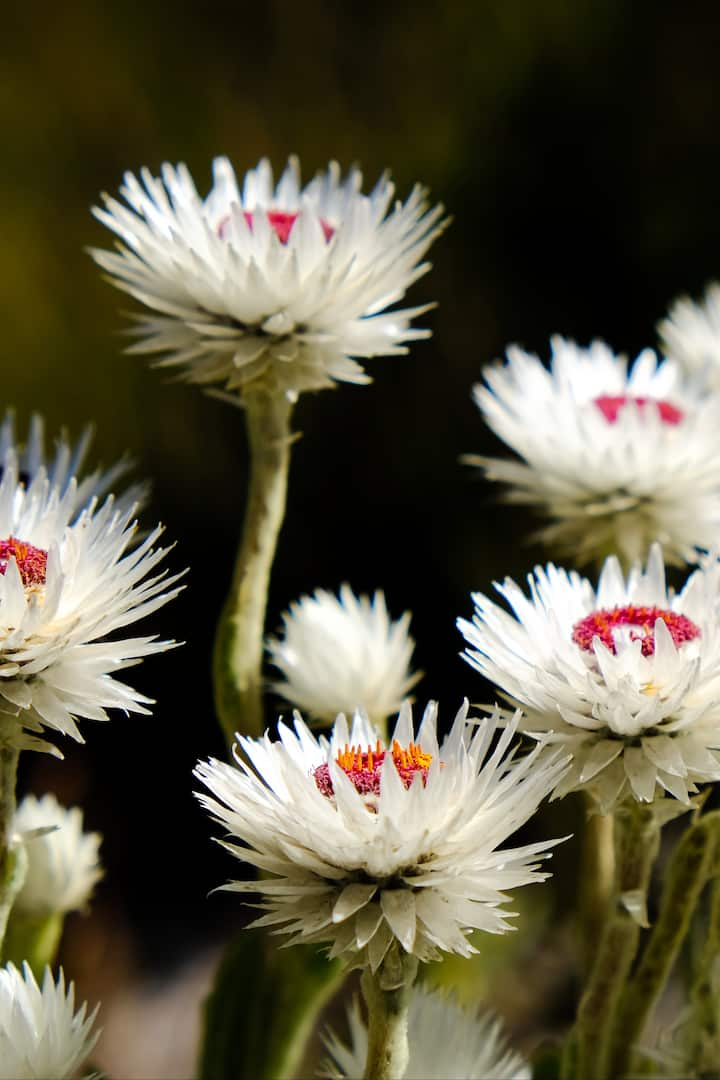This color photograph, captured in an outdoor setting, showcases a close-up view of approximately eight wildflowers against a dark green gradient background that transitions from a darker to a khaki green hue. Each flower, identical in appearance, features multiple rows of delicate white petals angling upwards around vibrant red centers. Some of the red centers present subtle hints of yellow stamens reaching upward. The flowers sit atop thick, asparagus-like light green stems. The tallest flower is positioned in the top left corner, while the others are asymmetrically arranged across the image, with a smaller one in the middle and several ranging from the bottom right-hand corner to the top right-hand corner. Among them is one flower turned away from the camera, obscuring its center. The background includes several small buds that remain unopened, complementing the overall composition of this realistic and finely detailed photographic representation.